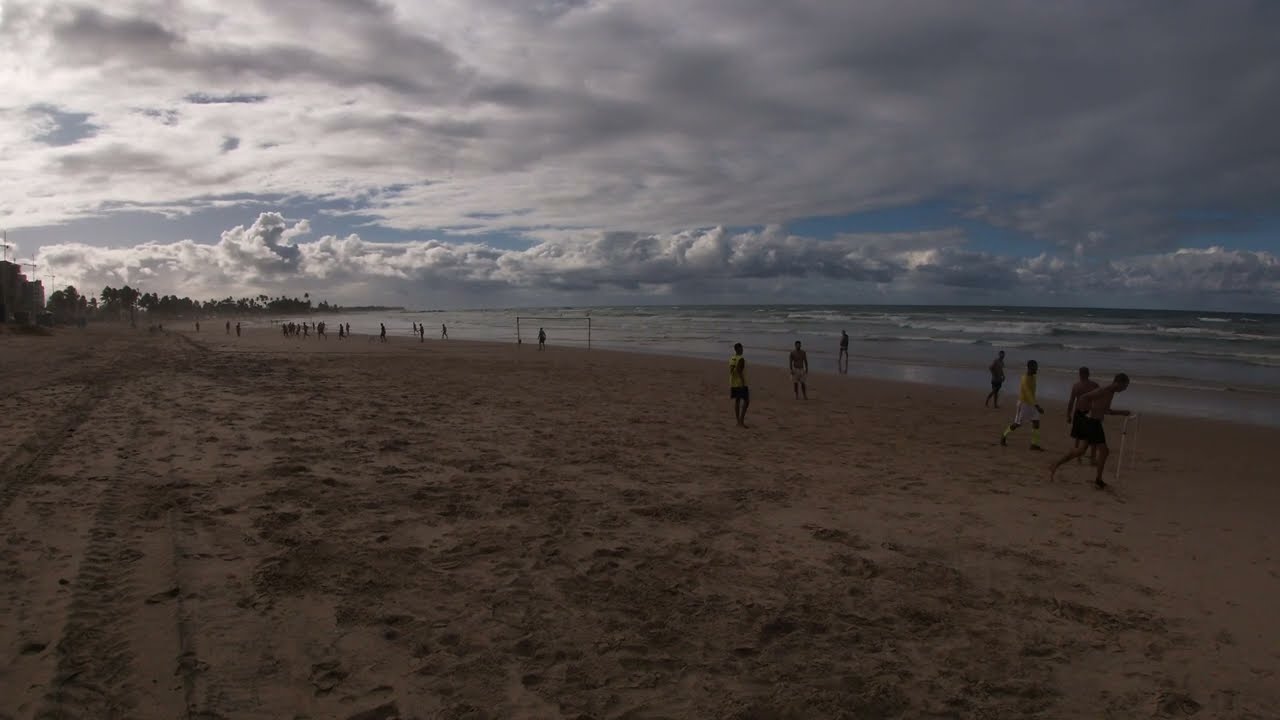The image captures a dusky beach scene where the setting sun, partially obscured by clouds and the horizon, casts a dim and moody light over the landscape. The sky is a dark blue with a patchwork of light and dark gray clouds that appear almost within reach. The focal point is a heavily churned sand area, filled with hundreds of footprints, indicating recent activity. The ocean to the right has a grayish tinge, blending seamlessly with the overcast sky. In the distance, whitecaps are visible amid the waves. 

At the center of the image is a goal light structure, suggesting an impromptu game of beach soccer. Multiple people, mostly in shorts and either shirtless or wearing short sleeve shirts, are seen walking or running towards the right side of the image. Notably, one individual in a yellow shirt and white shorts is running in that direction. Along the water's edge, people stretch towards the far back of the image, adding to the lively yet serene atmosphere of the scene.